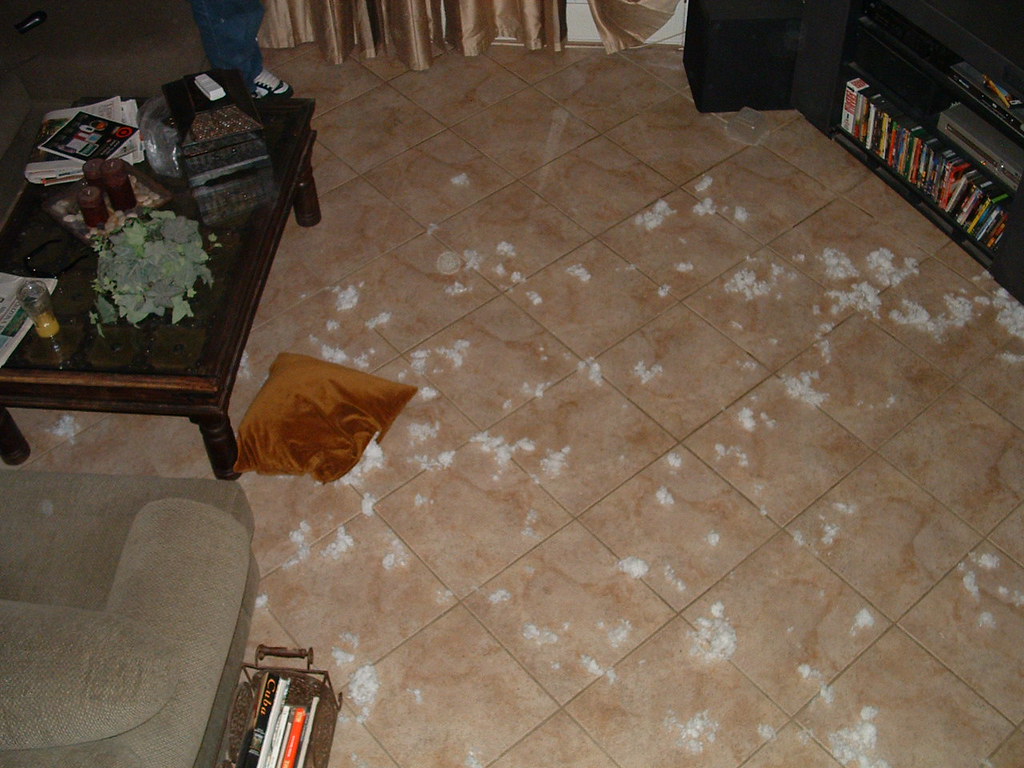In the image, a scene of domestic disarray is captured on a tiled floor, which has a pale brown hue. The main focus is a dark brown cushion that has been ripped open, spilling its stuffing onto the floor. This haphazard spread covers much of the floor, except for a small area near the top center. To the top right, there is an entertainment center, housing a TV, with a VCR and DVD player beneath it, and multiple DVD cases arranged vertically below. On the left side of the image, there is a small table positioned beside a grayish sofa. The table is cluttered with various items, including a white remote sitting atop a small lock case, a newspaper in the top right corner, a plant on the bottom right, and some candles. A person, partially out of frame, stands in the top left corner, identifiable by their jeans and shoes.